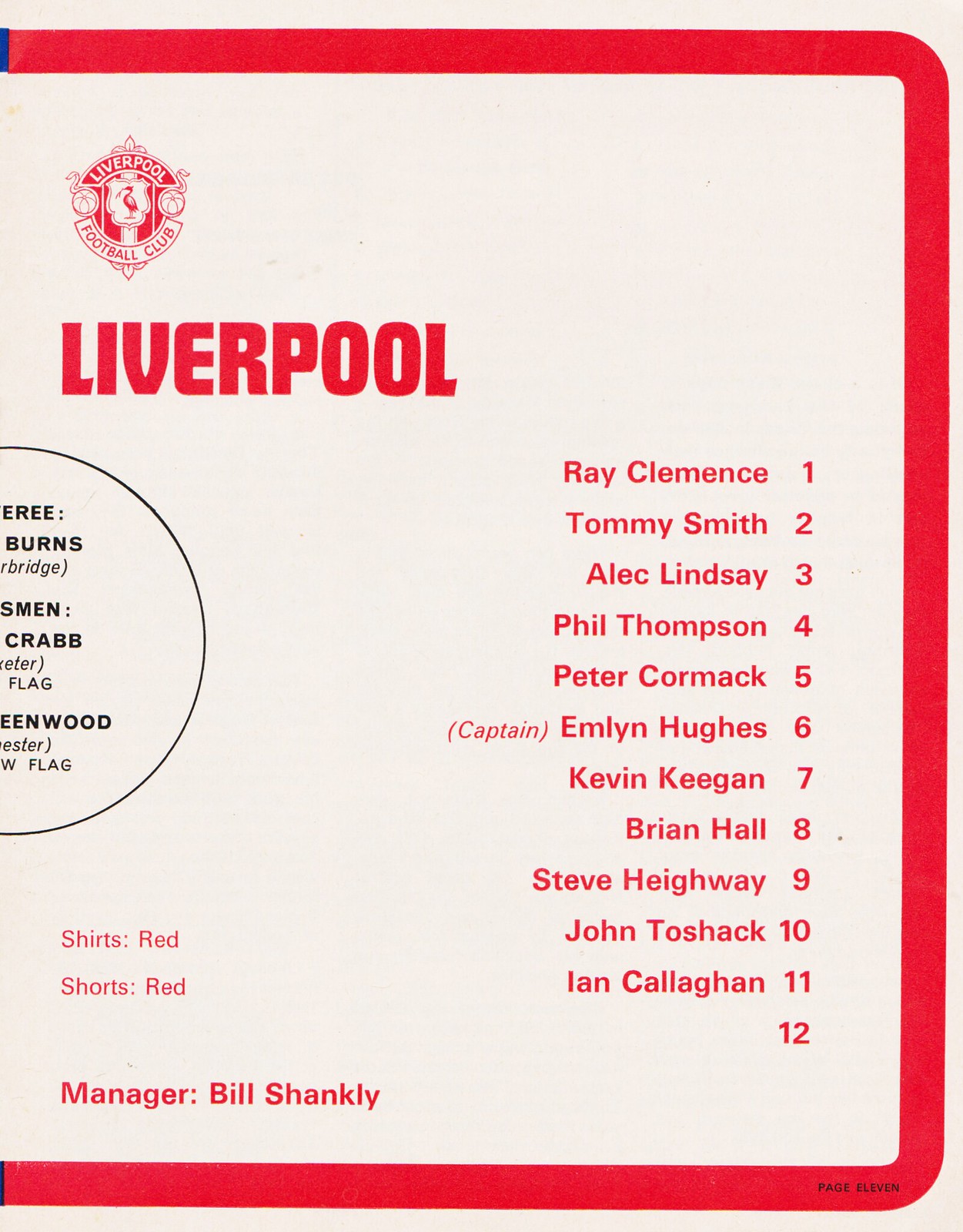The cover of this sports program or magazine features a solid white background framed by a thick red border around the edges. Prominently displayed on the upper left is a logo for the Liverpool Football Club, beneath which the word "Liverpool" is written in bold red text. Adjacent to this, there is a half-visible circle on the left side with partially obscured black text. The right side of the cover lists team members in a column with each player's name paired with their corresponding number: Ray Clements (1), Tommy Smith (2), Alec Lindsay (3), Phil Thompson (4), Peter Cormack (5), Captain Emlyn Hughes (6), Kevin Keegan (7), Brian Hall (8), Steve Heighway (9), John Toshack (10), and Ian Callaghan (11), followed by the number 12 without a name. The bottom left corner includes the details "Manager Bill Shankly" and above it, "Shirts Red, Shorts Red" in red text. Overall, the design is clean and structured, emphasizing the iconic red colors associated with the team.